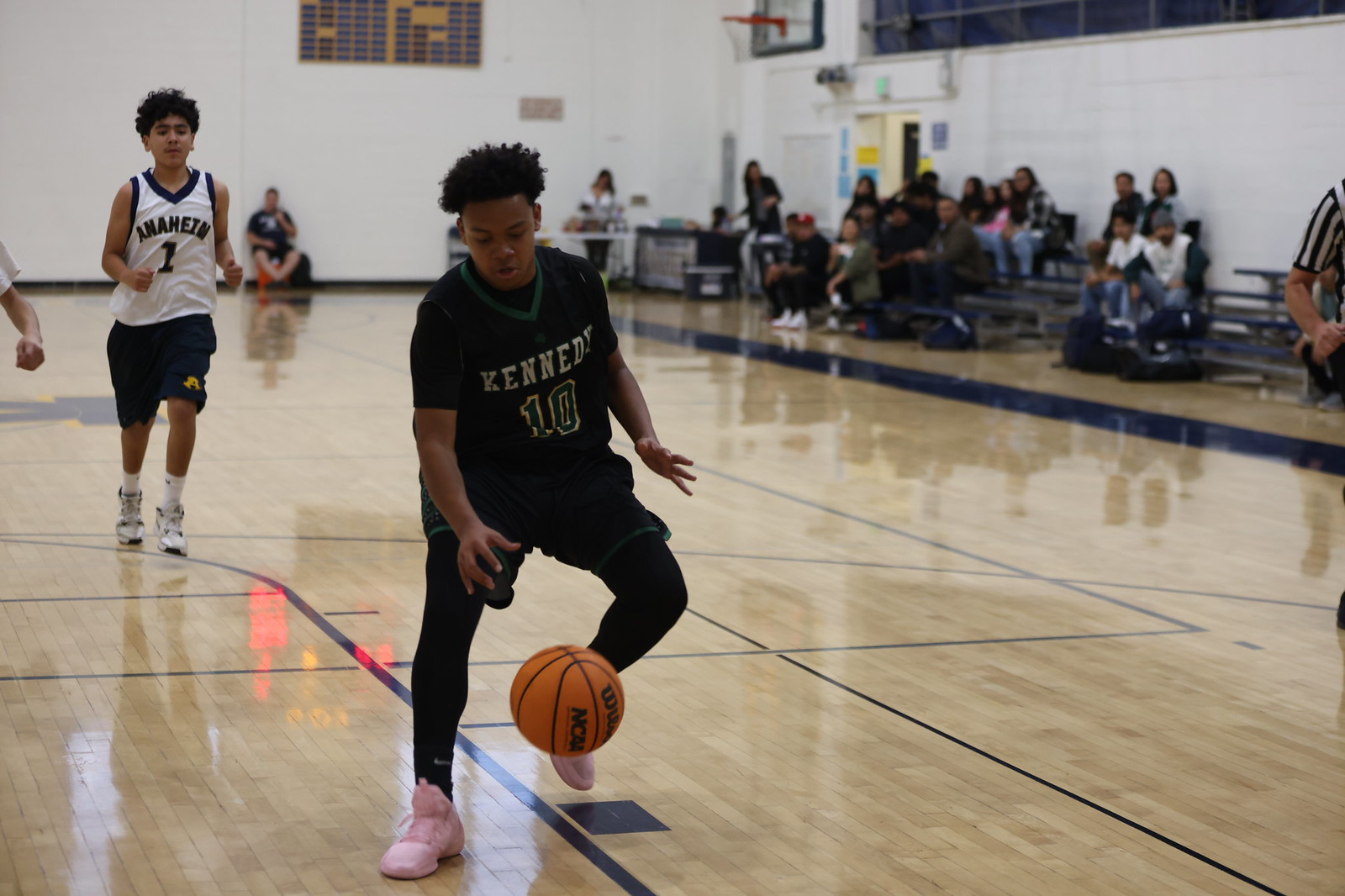The image captures an indoor high school basketball game in progress. The central figure is a young player from the team "Kennedy," wearing a black jersey with white text reading "Kennedy" and the number 10 displayed in green with yellow borders. The player, who appears intensely focused on dribbling the basketball, is outfitted in black leg compression stockings, long black pants, short green shorts, and bright pink shoes with pink laces. The polished, reflective light brown wood basketball court features multiple blue lines designating areas of play. In the background, another player from the opposing team "Anaheim" is visible, wearing a white jersey with the number 1 and dark blue shorts. The gymnasium's setting includes white cinder block walls and large windows in the top right corner, with bleachers along the far right wall occupied by onlookers.